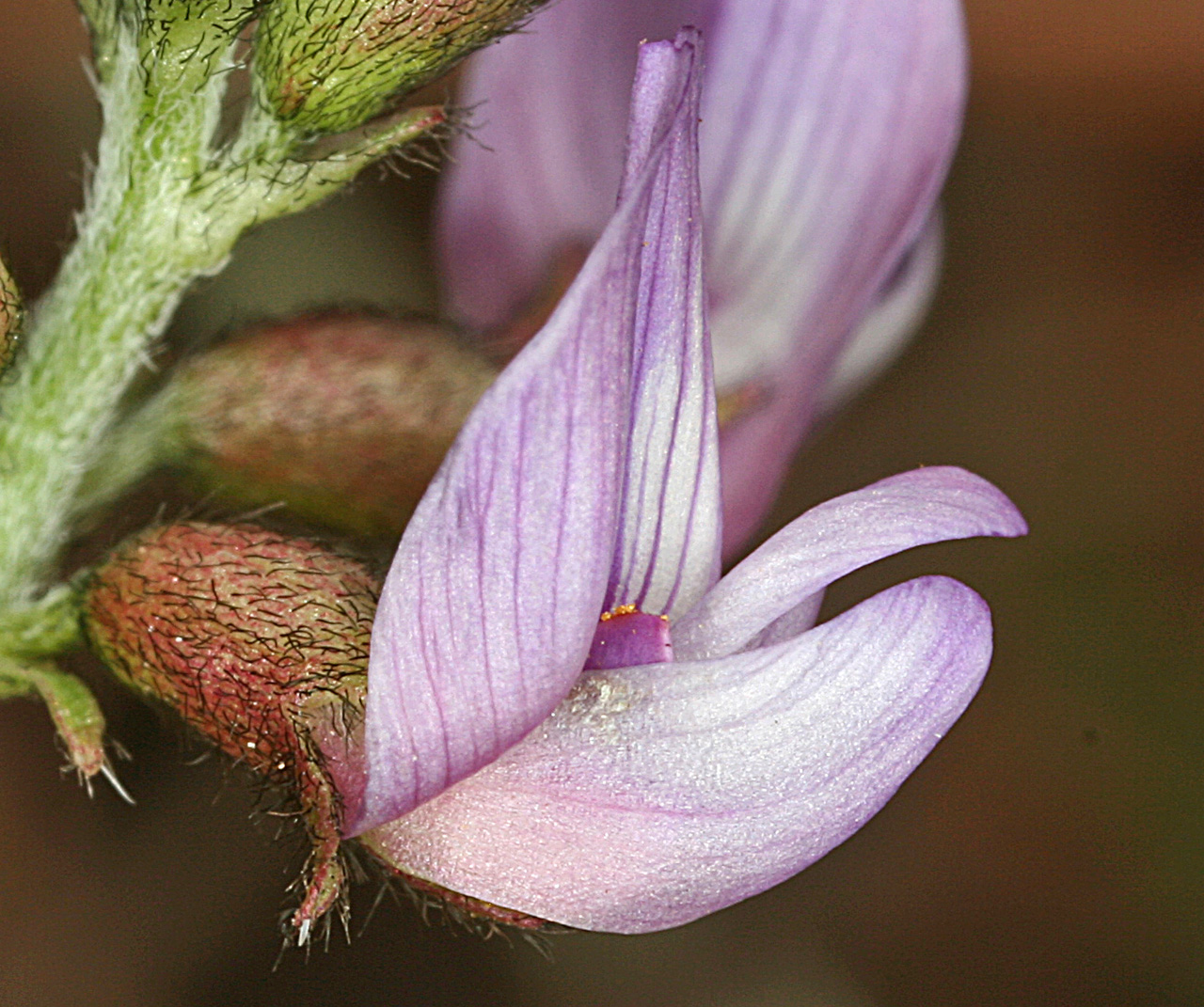This horizontal photograph showcases a close-up of a partially blooming purple flower that is possibly a snapdragon, captured in vivid detail. The main flower, prominently displayed in the center, features a combination of unopened and opened petals. The petals that are opening up are primarily purple with darker purple veins, forming an L shape with one spade-shaped petal pointing upward and another triangular petal pointing to the right. The flower's center appears to be a deeper purple hue with subtle yellow specks.

The base of the flower exhibits a reddish-green color adorned with small, dark hairs or fibers, which also cover the stem. This green stem, situated in the left-hand corner of the image, rises upward and to the right, connecting to other flower bulbs displaying similar red and green tints covered in tiny black hairs.

In the background, there's another purple flower on the same stem, blurred and out of focus. The overall background is a mix of unfocused brown and orange hues, creating a soft, ambient contrast that highlights the sharp details of the blooming flower in the foreground.